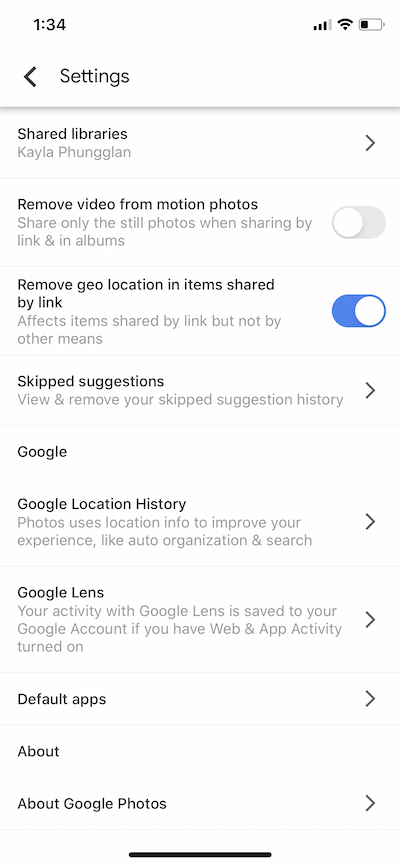A detailed caption for the image:

"The screen displays various advanced settings within the Google Photos app on a smartphone. Visible options include 'Shared Libraries' and a user named 'Kayla Phunglan.' Among the settings, there are toggles for removing videos from motion photos and geolocation data from items shared by link. Other options such as 'Google Location History,' 'Google Lens,' 'Default apps,' and 'About Google Photos' are also accessible. Users can manage metadata and location services, deciding whether to enable or disable these features. Additionally, there's an option to view and remove skipped suggestion history, and control the activity saved to their Google account related to Google Lens usage."